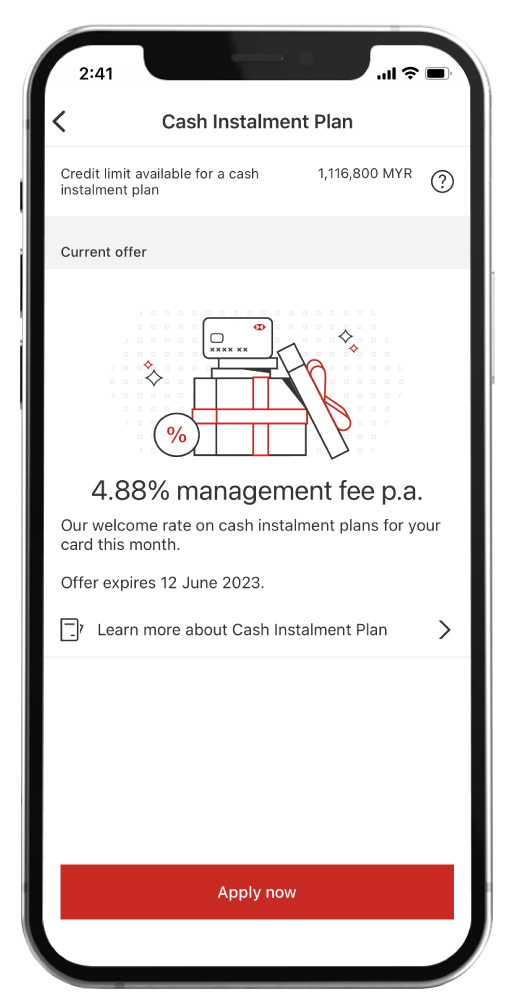The image is a portrait-mode digital illustration of a cell phone displaying a screenshot. The phone outline features a small button on the left side, beneath which are two larger buttons. At the upper left-hand corner of the screen, the numbers "241" are visible, while the upper right-hand corner shows a battery charge of approximately 75%.

The next row of the screenshot contains the text "Cash INSTALMENT plan," with "Installment" incorrectly spelled. A back arrow is present on this row as well. Following this, there is information about the available credit limit for a cash installment plan, again with "Installment" misspelled. The available limit is specified as "1,116,800 MYR," accompanied by a question mark icon.

Below this, a gray background section displays the heading "Current Offer." Within this section is an image of a gift box containing a gift card along with a percentage sign. The text reads: "4.88% management fee PA. Our welcome rate on installment plans for your card this month. Offer expires 12 June 2023. Learn more about cash installment plan."

At the bottom of the screen, a large red button is visible, although most of it is blank space. In small font within this button, the words "Apply Now" are written.